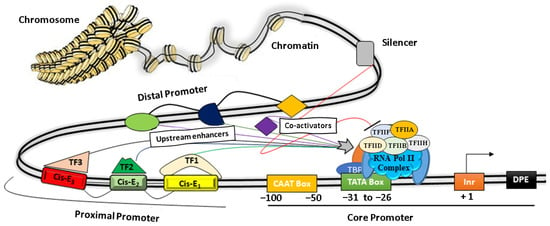This detailed image is a color infographic from a chemistry book, illustrating the structure and components of a chromosome, RNA, DNA, and related bodily functions. The background is white, and the diagram is in a landscape orientation. On the top left, labeled in black text, is the word "chromosome" next to a beige, bottle-brush-like structure with black outlines, which curves in a backward 'S' formation. 

This curve features a yellow honeycomb cell pattern with black stripes, resembling a spiral tube with discs along the curves. Various labels in black text along the structure outline terms like "chromatid," "chromatin," and several key genetic components.

As the curve progresses to the right and downwards, it incorporates an array of horizontal rectangles in diverse colors, representing different elements such as "silencer," "distal promoter," "proximal promoter," and "core promoter." Each of these components is color-coded with green circles, blue half-circles, yellow squares, and purple squares. 

Above the proximal and core promoters, there are mini diagrams with black squares and rectangle shapes in red, green, yellow, orange, brown, and black. These mini diagrams include labels like "DPE," "CAAT box," "TATA box," "TFIID," and "TFIIB." A measurement bar ranging from -100 to +2 is displayed below these elements, featuring markers at -100, -50, -31, -26, -2, -1, and +2.